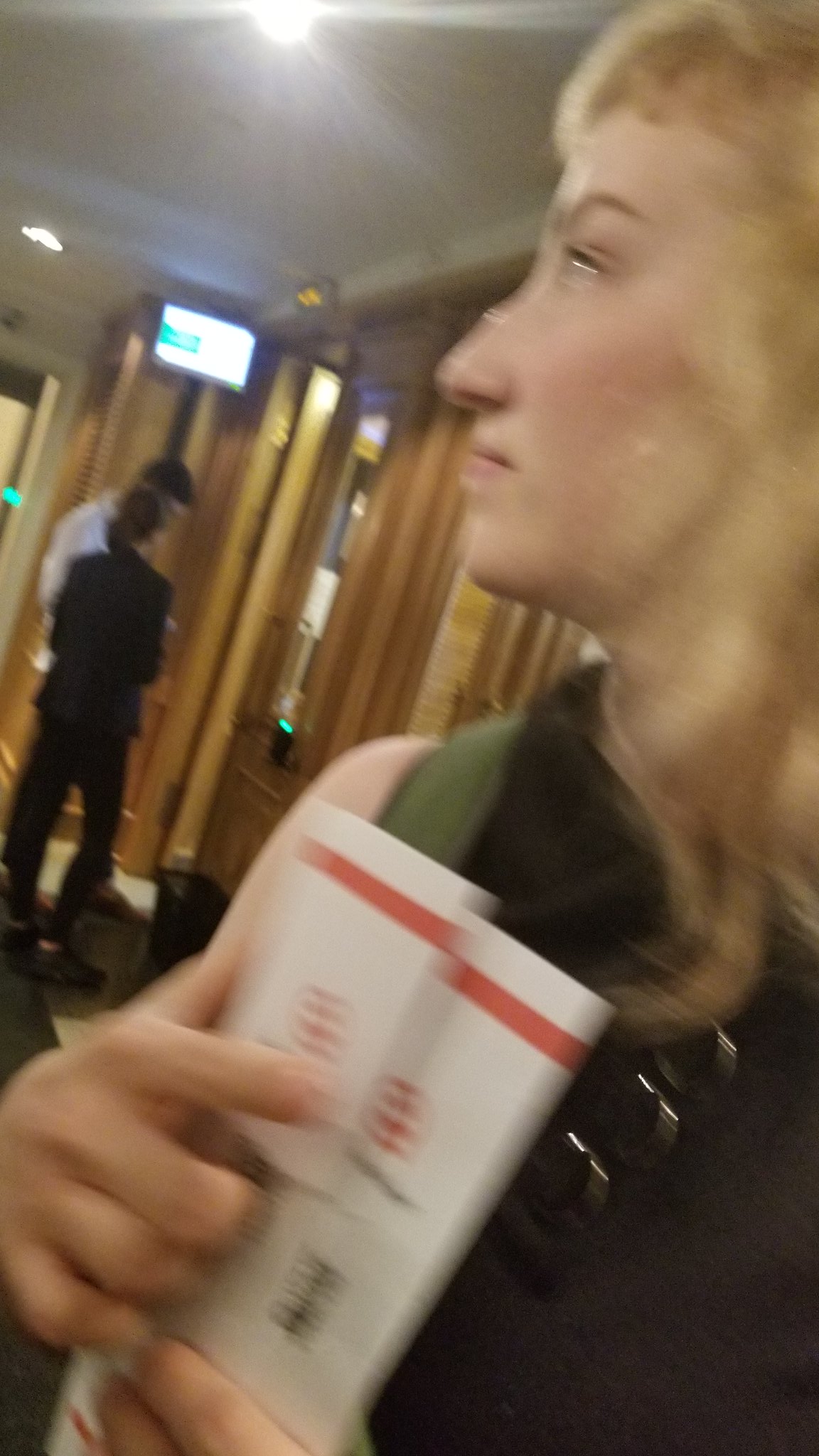This color photograph, slightly blurry and out of focus, captures a candid moment. In the upper right-hand corner, the side profile of a pale-skinned white woman with blonde hair that falls just below her shoulders is visible. She is dressed in a sleeveless green shirt, revealing a portion of her right shoulder. In the lower left-hand corner, her right hand can be seen holding a couple of books or brochures, each featuring a distinctive red stripe at the top. The backdrop suggests an interior setting, likely a gym, where two men are faintly seen near a weight machine, though the details are blurred and indistinct.